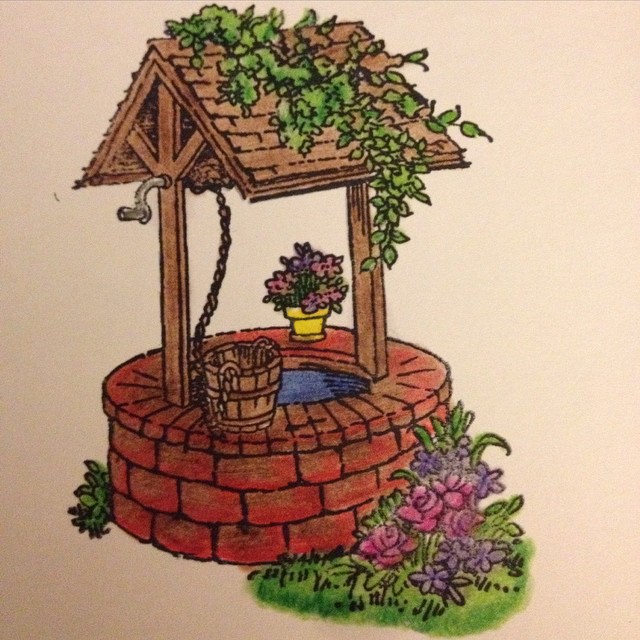This is a detailed drawing reminiscent of a storybook illustration, depicting a charming, round water well with a brick base. The lower portion of the well features large, reddish-brown bricks, while the top is built with smaller bricks. Supporting the well is a traditional wooden structure capped with a shingled, angled roof, partly covered in creeping ivy. A silver crank handle, situated on the left side beneath the roof, winds a chain connected to a wooden bucket that rests at the well's edge. Beside the bucket, on the right side, there is a yellow flower pot brimming with vibrant pink and purple flowers, highlighted by numerous green stems. Additional flowers in shades of purple and pink, along with patches of green grass, adorn the foreground and surround the well, completing this picturesque scene. The entire background is a warm, welcoming pink.